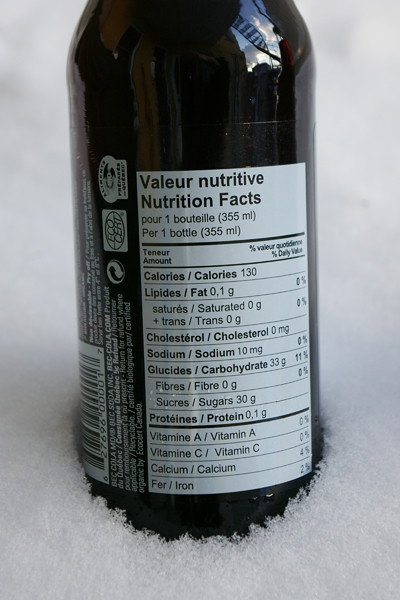The photograph features an extreme close-up of a bottle sitting in a pure white snowy or fine ice crystal texture, suggesting either a winter setting or a cooler environment. The bottle, made of dark transparent glass, is so opaque that its contents remain unseen. The focus is on a white label with black text displaying nutritional facts, prominently positioned towards the camera, obscuring the identity of the product. The label includes information in both English and French. Details such as "Valero Nutritive," the serving size of "one bottle, 355 milliliters," and specific nutritional values like "calories, 130" and other daily values are clearly readable. The surrounding ice crystals are visible around the bottom edge of the bottle, enhancing the cold, pristine setting of the image.